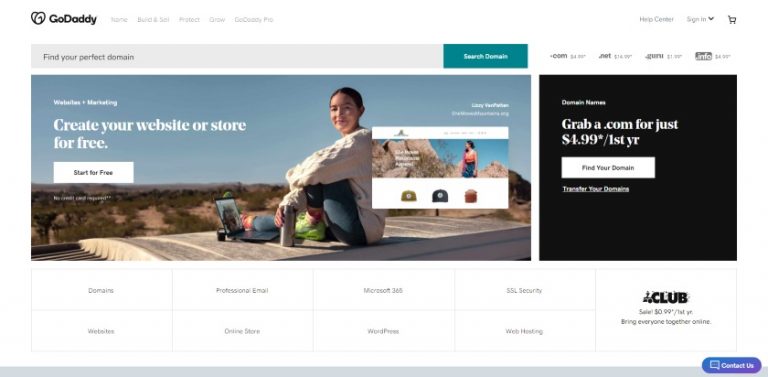This screen capture showcases the GoDaddy website, meticulously organized into distinct sections for user convenience. 

At the top of the screen, a comprehensive menu bar offers various navigation options, including account management and cart access. Just below, a prominent search bar labeled "Find Your Perfect Domain" invites users to search for domain names, supported by adjacent instructional text.

The central portion of the screen is dominated by a visually engaging image depicting a woman seated atop a camper, evoking a sense of adventure and freedom. This area, extending approximately two-thirds across the screen, features several interactive elements such as text and choice bars, enhancing user engagement.

To the right, a vertically aligned section occupies about one-third of the screen, providing additional contextual content or options.

Below the central image and interactive area, multiple buttons facilitate user actions, seamlessly leading into a concluding gray bar. This bar is complemented by a prominent blue button with white text reading "Contact Us," ensuring easy access to customer support.

Overall, the design cohesively presents GoDaddy's offerings, emphasizing the ease of starting a domain search or taking advantage of special offers like obtaining a .com domain for just $4.99 for the first year.